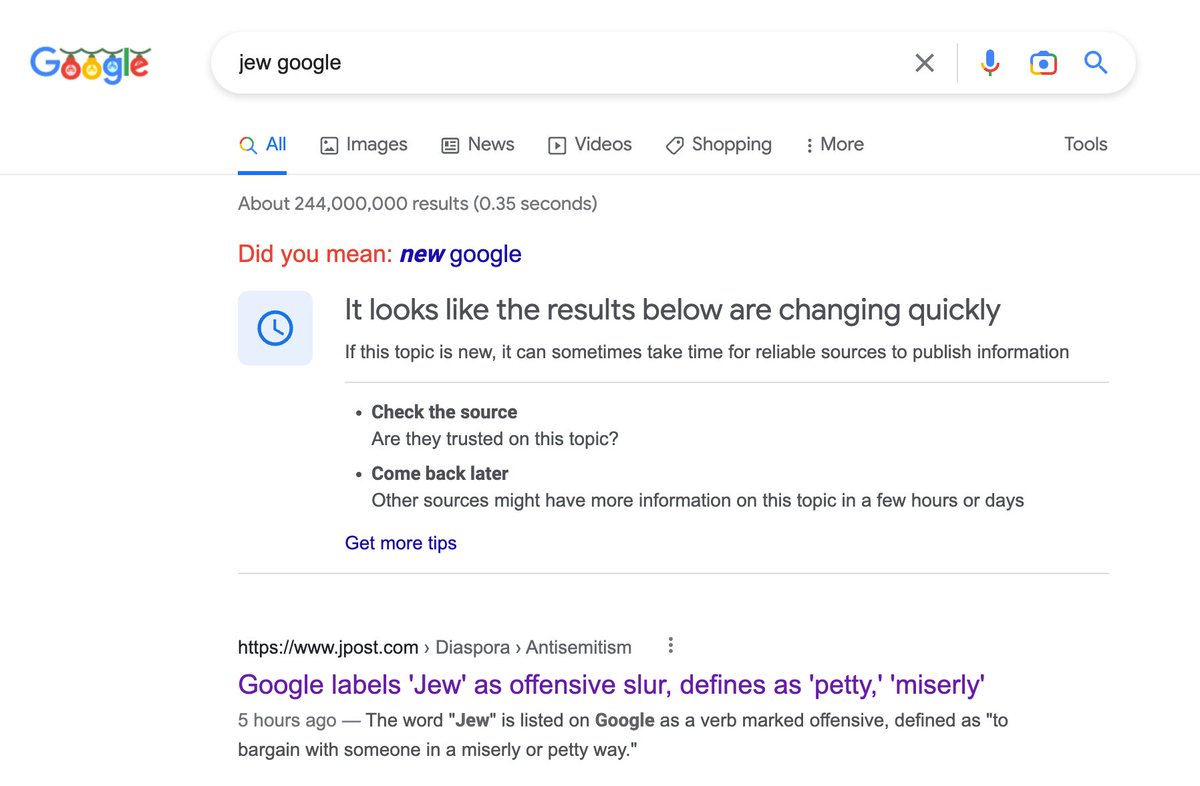The image depicts a Google search results page featuring the colorful Google logo in the top left corner, which is styled as a string of Christmas lights with the word "Google" hanging down. To the right is the familiar white search bar, displaying the search query "Jew Google." The "All" tab is selected and underlined in blue. 

A notification bar below the search tabs states, "It looks like the results below are changing quickly. If this topic is new, it can sometimes take time for reliable sources to publish information." A small blue square with a clock icon appears next to this message, alongside advice to "check the source. Are they trusted on this topic?" and a suggestion to "come back later or other sources might have more information on this topic in a few hours or days." 

Further down, a purple link reads, "Get more tips." Below a gray divider line, a search result is shown from the website "https://www.jpost.com," under the category "diaspora antisemitism." The link, in purple text, says, "Google labels 'Jew' as offensive slur, defines as petty miserly." The description clarifies, "Five hours ago, the word 'Jew' is listed on Google as a verb marked offensive, defined as to bargain with someone in a miserly or petty way."